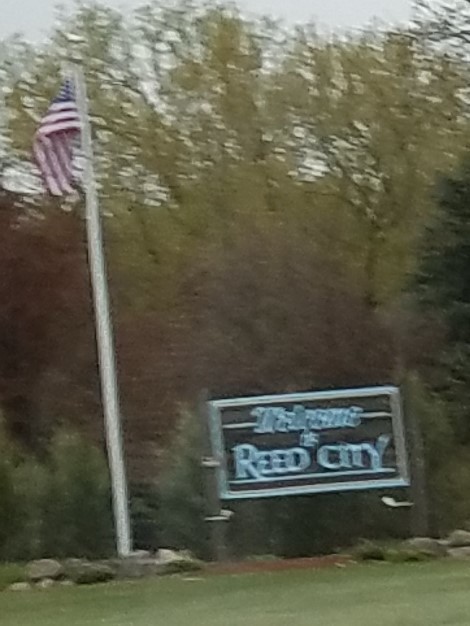This photograph captures an outdoor scene featuring a welcome sign for Reed City. The sign, composed of white script lettering adorned with an underline and painted on a wooden, brown background, reads "Welcome to Reed City" in capital letters. To the left of the sign stands a prominent white flagpole topped with a silver finial, hoisting an American flag resplendent in red, white, and blue. Surrounding the base of the flagpole and sign are various large rocks and patches of green grass. In the background, a stand of trees with a mix of dark red and green foliage forms a natural backdrop, although the entire image appears slightly out of focus, lending a blurry, low-quality appearance to the scene. The sky, in a grayish hue, peeks through the canopy of trees, further enhancing the rustic and welcoming atmosphere of Reed City.